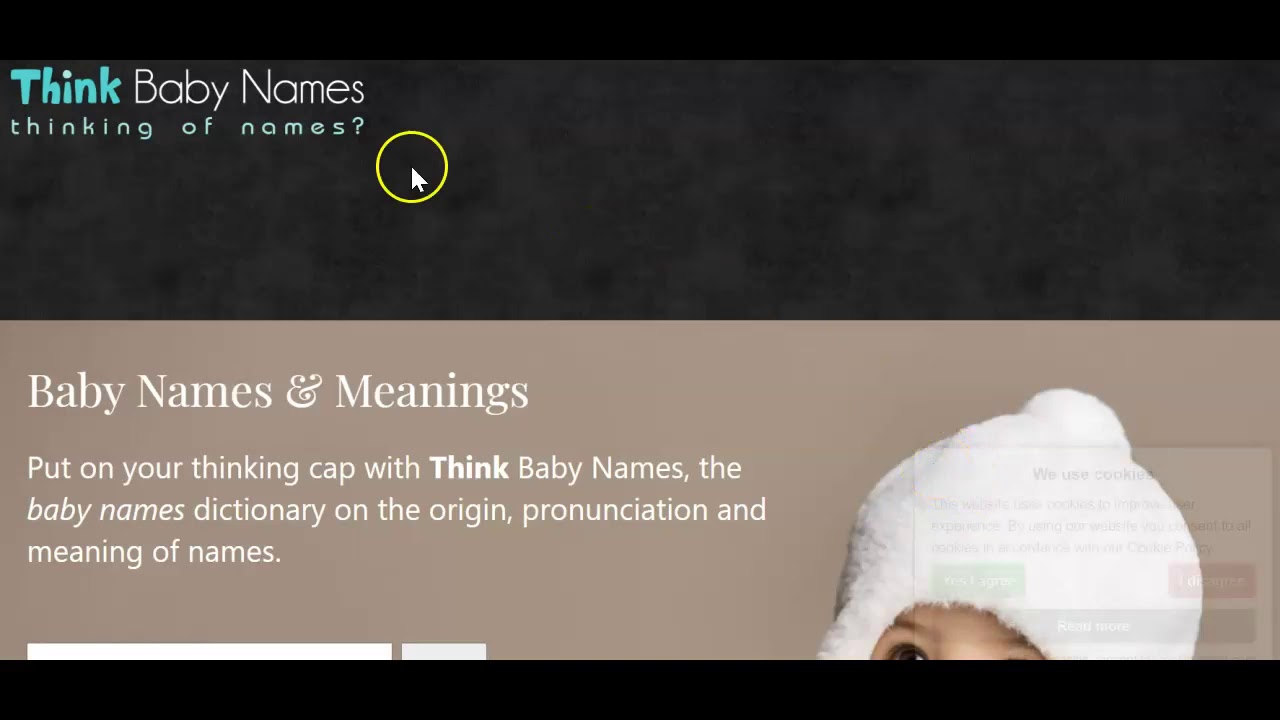The image displays a desktop screenshot of a website with a sophisticated black and tan color scheme. The top section of the screenshot features a thin black bar along the very top, followed by a black and gray gradient background. In the upper left corner, the text "Think Baby Names" appears in a playful round font. The word "Think" stands out, being shaded thickly and unevenly in a bluish-green hue. A neon circle surrounds the cursor on the screen, drawing attention.

The lower half of the screen transitions to a tan background, prominently displaying white text that reads, "Baby Names and Meanings. Put on your thinking cap with Think Baby Names, the Baby Names Dictionary on the origin, pronunciation, and meaning of names." To the right of this text, a cut-off photo of a baby's head is visible. The baby wears a thick, fuzzy white hat with ear flaps extending down the sides and a poof ball on top. Only the bridge of the baby's nose, its right eye and eyebrow, and its left eyebrow peeking out from under the hat are visible. Completing the composition, a black bar runs along the bottom of the screenshot.